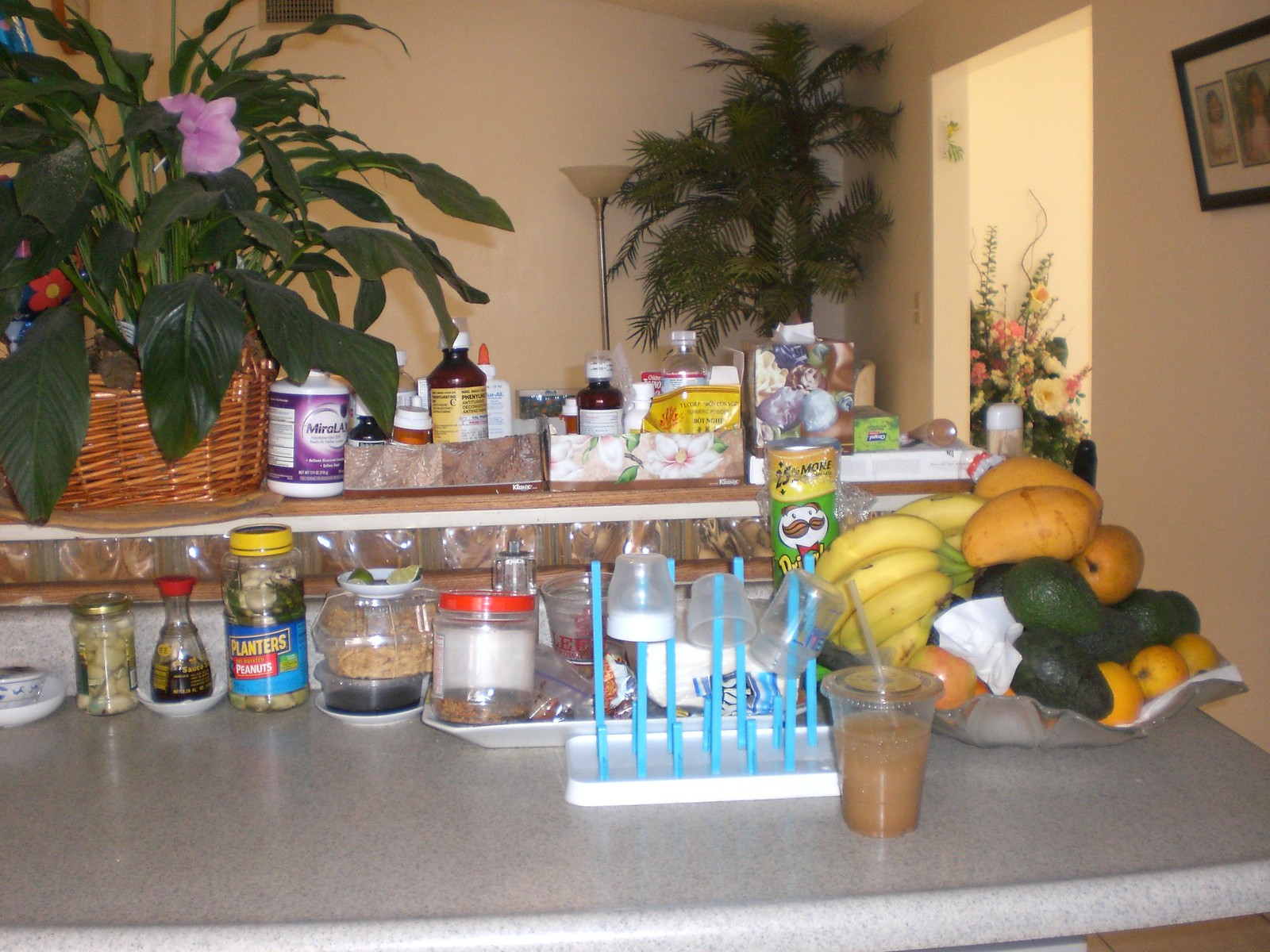In this detailed and bustling kitchen scene, every corner and surface tells a story. Toward the back, a tall palm tree stands grandly beside an unlit floor lamp, adding a touch of greenery. The central focus is an island counter with a ledge, home to a plant in a brown wicker basket, showcasing a single pale purple flower. Gathered around the plant are various items: a bottle of Miralax, different medications turned away from view, a brown and white Kleenex box, a glue bottle, and another Kleenex box decorated with pale white flowers. Scattered near these are what appears to be cough syrup and a third Kleenex box lying on its side, accompanied by chewing gum, deodorant or Tic Tacs.

To the side, a door frame appears, beyond which a large flowering plant is visible. Despite its lifelike appearance, its mixed flower and leaf types suggest it might be an artificial arrangement. Closer to the viewer, at the front of the counter, sits a white teacup or soup cup, decorated with blue patterns, resting in a matching saucer. A jar filled with chunks of an unidentifiable substance, possibly garlic, sits beside Kikkoman soy sauce in its distinctive bottle with a red lid. A Planters Peanuts jar, now repurposed to store what looks like mushroom tops, stands nearby.

Also present is a to-go container, probably holding ramen, and a small white plate with lime wedges atop it. Nearby, a container, potentially once filled with peanut butter, holds an unknown substance. Various takeout containers, a white package of napkins, a green container of Pringles, and a bowl filled with bananas, lemons, and a papaya or another similarly sized fruit, add to the clutter. The front of the image features a white tray functioning as a drying rack for baby bottles, with some bottle parts drying on it. Next to it rests a clear to-go cup with a pale-colored iced coffee.

The sheer number and variety of items suggest a kitchen in a small space, with limited room leading to an organized chaos. Each item tells a part of this kitchen’s active story, highlighting a mix of everyday tasks, from meal preparation to baby care.